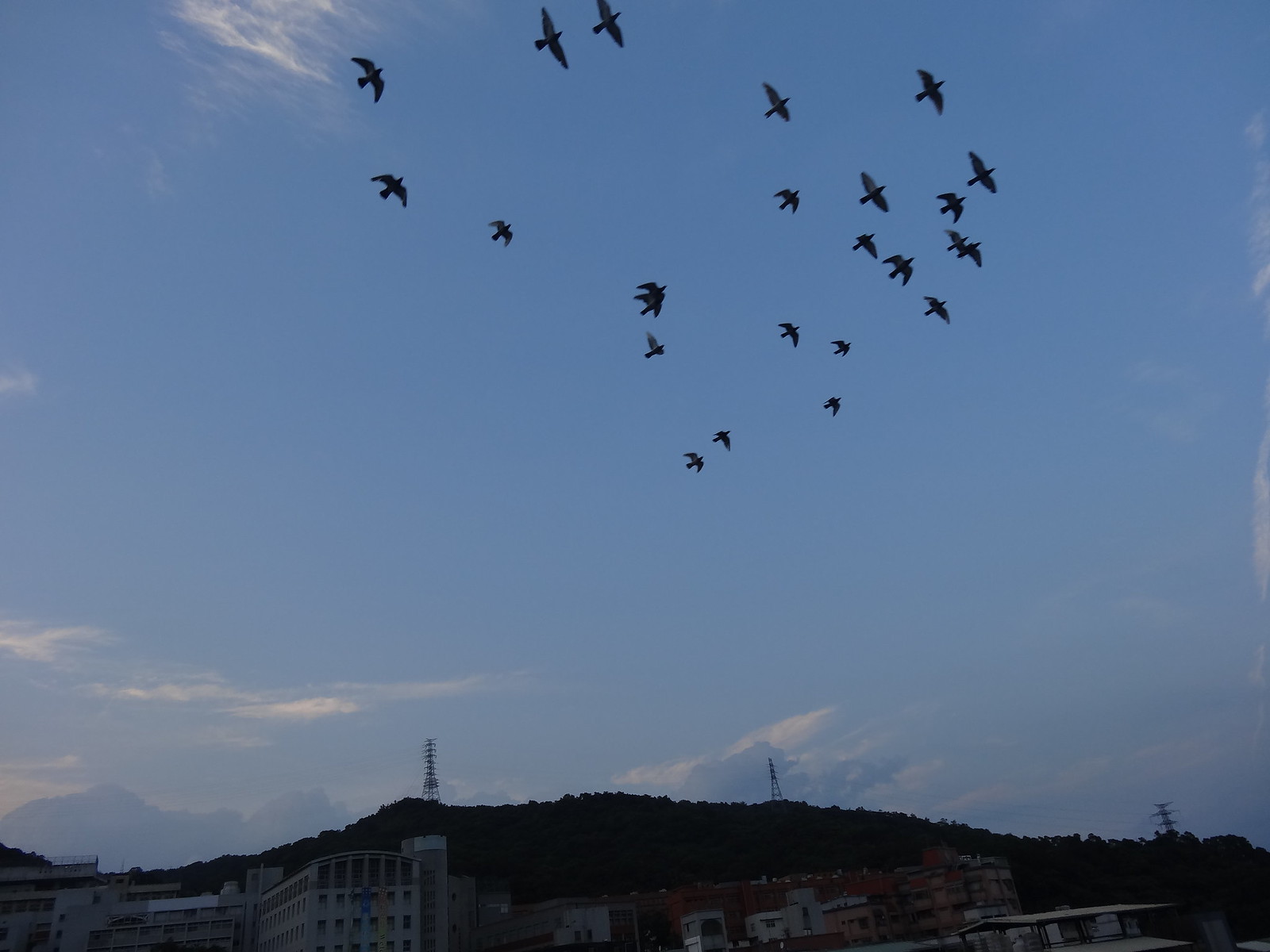Just before sundown, the photograph captures a scene looking up from the ground towards a darkening blue sky, where about two dozen seagulls are soaring in unison towards the upper right-hand corner of the image. They are set against a backdrop of both wispy white clouds and more substantial gray clouds on the horizon, signaling the imminent sunset as the sun dips behind the lower clouds. Below this dynamic sky, a hillside rises, crowned with three conspicuous electrical towers. At the base of the hill, a cluster of multi-story buildings of various shapes and colors appears, though they are shadowed and difficult to distinguish precisely. The overall scene juxtaposes the vibrant movement of the birds against the static presence of the man-made structures and the natural landscape.